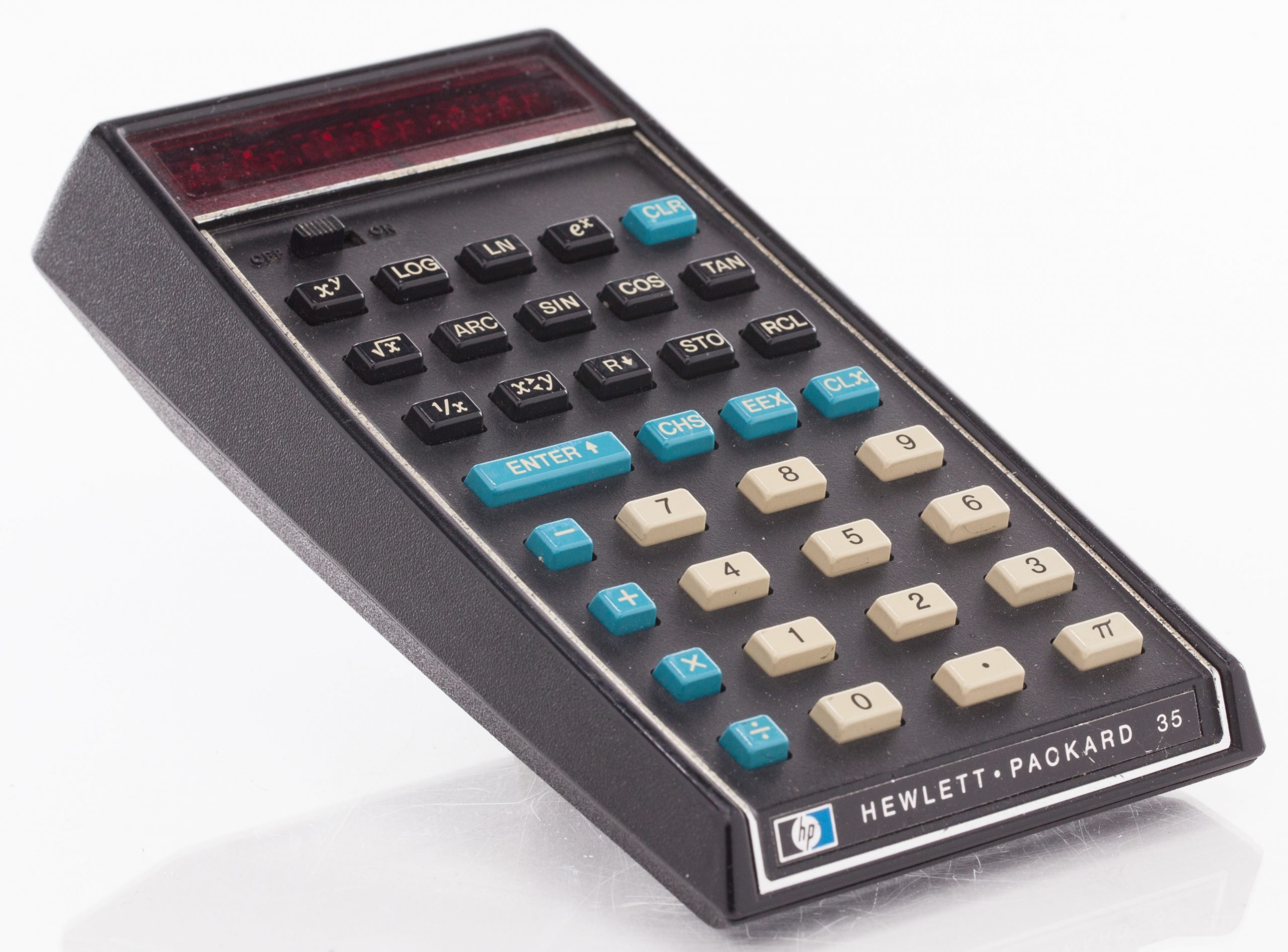This image features a close-up photograph of a Hewlett-Packard 35 scientific calculator, set against a white background. The HP 35, hailing from the 1970s or 80s, showcases an early predecessor to modern calculators with its rectangular, handheld design. The device is crafted from dark plastic, which appears either black or dark brown in different lighting. Dominating the top portion is an antique red LED display, a precursor to LCD screens. Among its multitude of functions are logarithmic calculations, exponents, and various trigonometric operations like sine, cosine, and tangent. The calculator is equipped with a sliding black on-off switch and an assortment of buttons: tan buttons for the numbers 0-9, light blue buttons for fundamental arithmetic operations such as addition, subtraction, multiplication, and division, as well as black buttons for advanced mathematical functions like square roots. The bottom of the device bears the distinct text "Hewlett-Packard 35" alongside the HP logo.